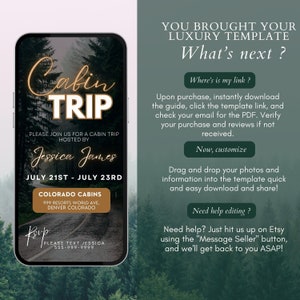An advertisement is split vertically down the middle, featuring a serene background of green trees and blue sky on both sides. On the left side of the ad, a prominent black rectangular shape stands out against the background. At the top of this black rectangle, the word "CABIN" is written in gold letters. Below it, the word "TRIP" appears in white letters. Additional gold text follows, and beneath that, the dates "July 21st through July 23rd" are displayed in white letters. At the bottom, "Colorado Cabins" is written in white letters on a brown background.

The right side of the ad mirrors the same background of green trees and sky but is tinted green. In white letters, it states, "You bought your luxury template. What's next?" Below this, additional white text guides the user with instructions: "Upon purchase, instantly download the guide. Check the template link and check your email for the PDF. Verify your purchase and review if not received." Further down, it instructs to "drag-and-drop your photos and information into a template, quick and easy. Download your template." At the very bottom, it reads, "Detailed just hit us up on Etsy using the message seller button and we'll get back to you ASAP."